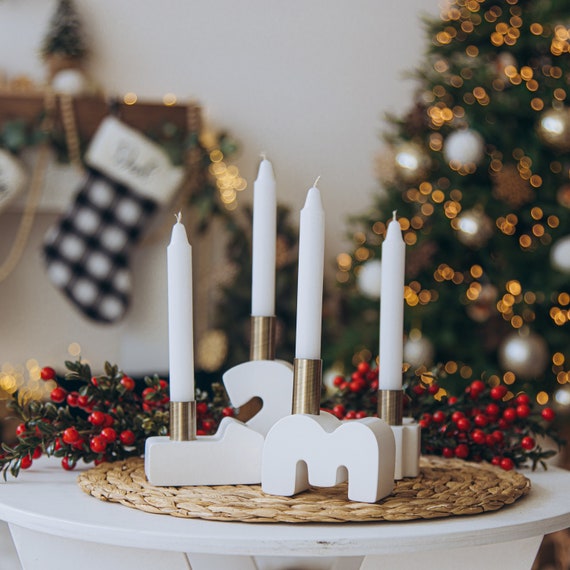This photograph, likely intended for a holiday catalog, captures a serene Christmas scene with a warm, festive ambiance. In the foreground, a set of four slender, unlit white taper candles are elegantly arranged in distinct votive candle holders. The holders resemble abstract numbers, suggesting a countdown or advent theme. These candles rest atop a round wicker placemat positioned on a white wooden table. Behind the candles, a meticulously arranged display of artificial cranberries and foliage adds a touch of classic holiday decor. 

The softly focused background accentuates the Christmas atmosphere with a decorated tree glowing with gold lights and silver ornaments on the right. To the left, a black-and-white buffalo plaid stocking hangs from a mantle, adding a cozy, personal touch to the setting. The bokeh effect enhances the warmth and festivity, making the image a perfect representation of a classic Christmas scene.